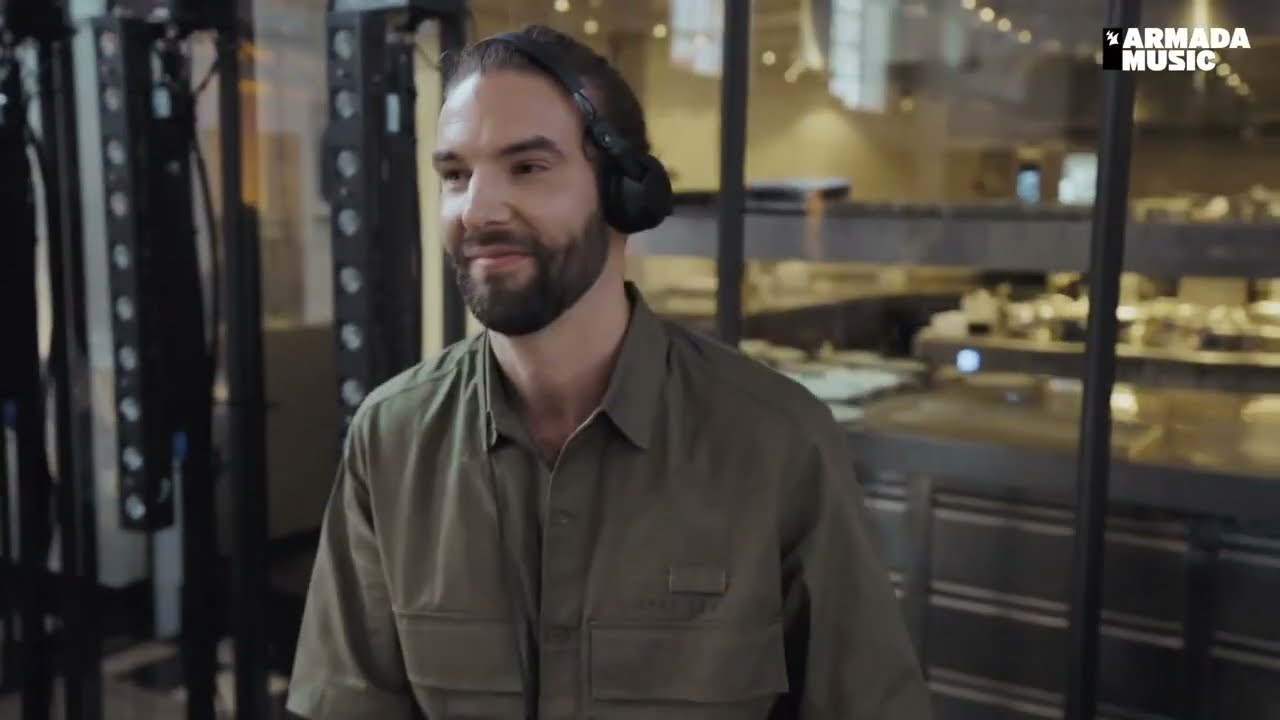The image features a man positioned at the center, sporting a dark green button-down shirt and black headphones over his ears. He has short brown hair and a well-groomed beard, with a mustache, both a dark brown color. The man is smiling gently, his head and gaze slightly turned to the left. Behind him, a glass or window pane framed with black bars is visible, hinting at an indoor setting, possibly a recording studio or office space. The room behind the glass is illuminated with yellow light, revealing tables, desks, and what might be a conveyor belt or workbenches. At the top right corner of the image, in bold white capital letters, is the text "Armada Music". The overall color palette includes shades of black, white, gray, tan, brown, dark green, olive green, light pink, off-white, yellow, and orange, contributing to a vibrant yet professional atmosphere.